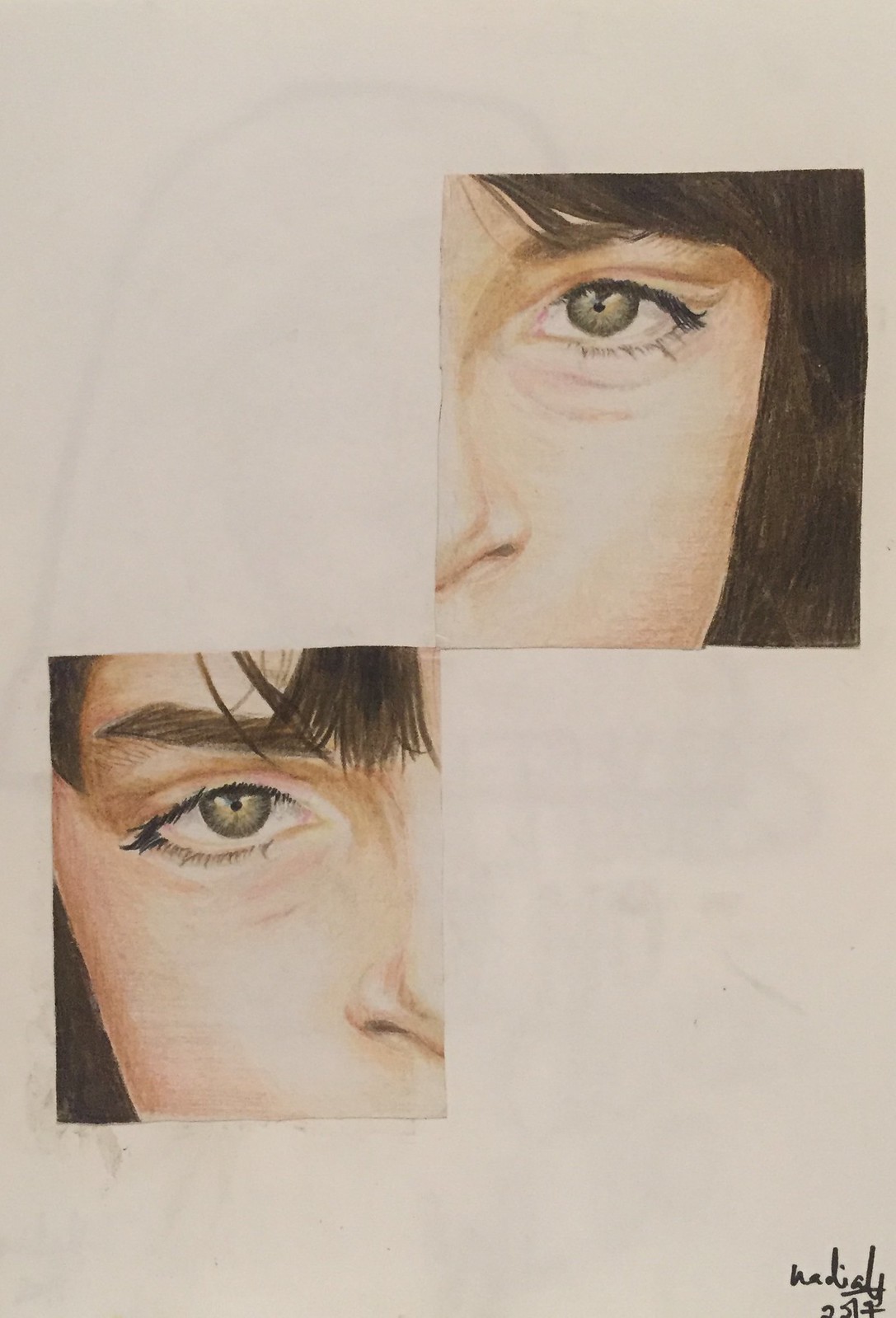In this colored pencil drawing by an artist whose signature appears to read "Nadialy" or "Madeline" in the bottom right-hand corner, we see a detailed depiction of a face split diagonally into two mirrored sections. The left-hand portion of the image features a green eye with brown eyebrows and black eyelashes. Visible are some bangs and a partial view of the nose. Diagonally opposite in the upper right-hand portion, the other eye shares the same green color, with matching brown eyebrows and black eyelashes. This side also shows more hair, highlighting the dark brown hair color, along with bangs and a complementary portion of the nose. Both sections of the face are framed by a white skin tone, forming a cohesive yet split representation of the same face, emphasizing symmetry and detail.